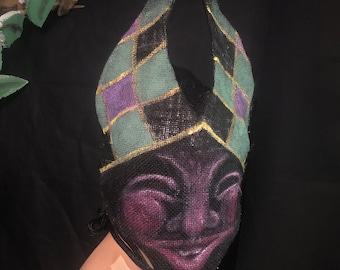An intricately detailed oil painting set against a stark black background portrays a person of color, possibly African-American, with purplish skin and squinted, smiling eyes. The individual is dressed in an elaborate headpiece that extends about six inches above the forehead, featuring designs in alternating squares of green, black, and purple, accented with gold, and adorned with dark green patterns resembling a fish. The headpiece splits into points, creating a horn-like effect, and they also wear a robe that appears to be either green, orange, or brown. In the foreground, green leaves peek into the scene from the left-hand corner, though the tight crop of the image obscures the broader context and additional details of the artwork.